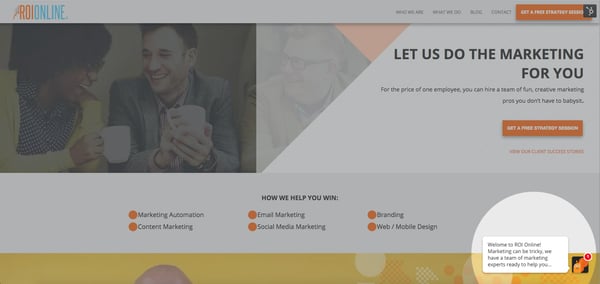The image displays a web page with a predominantly gray background. In the upper left-hand corner, the text "ROI Online" is clearly visible. The upper right section of the page contains blurry text. Despite the poor legibility, it appears to read: "What We Are," "What We Do," followed by an indistinct line, and then "Contact." In the very upper right-hand corner, set against an orange background, the text "Get A Free" is visible, but the rest of the message is blurred and unreadable.

In the main body of the page, there is black text on the gray background that boldly declares: "LET US DO THE MARKETING FOR YOU." This message emphasizes, "For the price of one employee, you can hire a team of fun, creative marketing pros you don't have to babysit." Below this statement, an orange banner reads "Get A Free," followed by mostly illegible text, except for the word "Session." There is also some additional text in orange below this, which remains blurry and unreadable.

On the far left side of the web page, a cheerful image captures a woman and a man sitting together, smiling and laughing while holding coffee cups. A third person, another man, is partially visible on the far right of the picture. Adjacent to this image, the text lists the services provided: "How We Help You Win: Marketing Automation, Content Marketing, Email Marketing, Social Media Marketing, Branding, Web/Mobile Design."